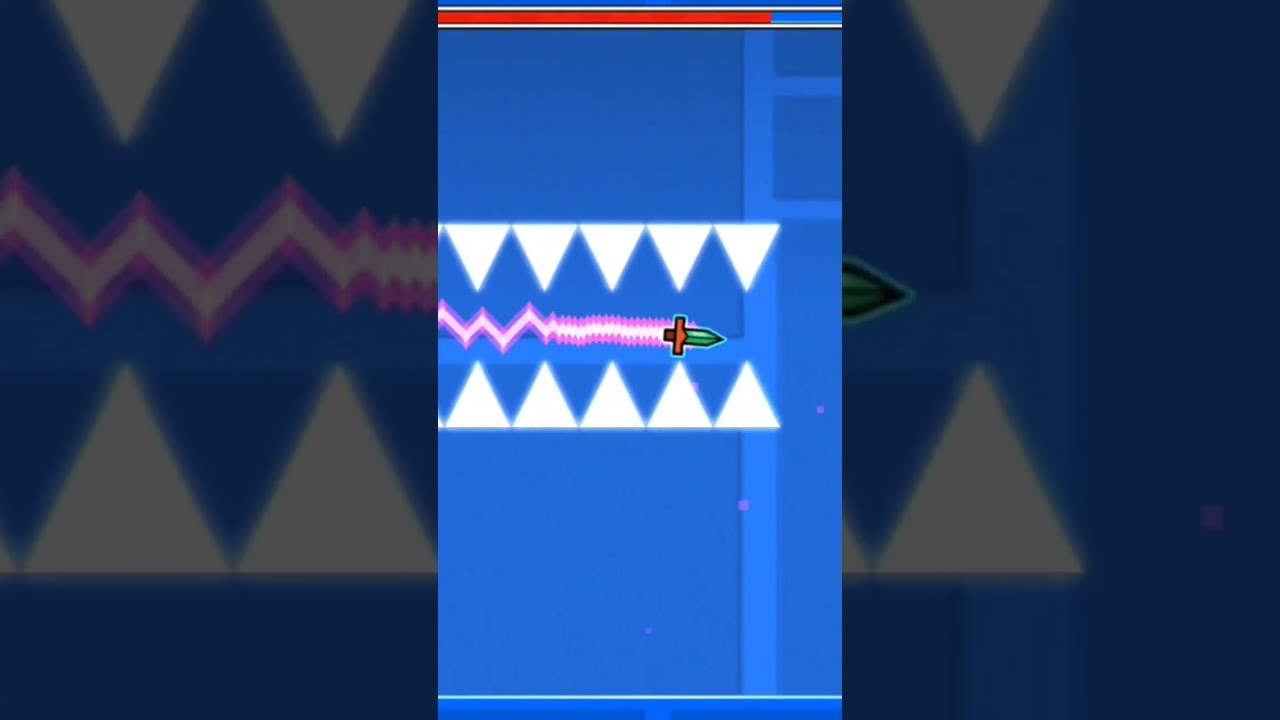The image appears to be a screenshot from a mobile video game featuring vivid and geometric graphics. Dominating the center is a tall blue rectangle, representing the primary game interface. At the top of this rectangle is a red progress bar, nearly 85% complete, framed by thin horizontal pinstripes. The sides of this blue rectangle are bordered by white frames divided into smaller sections, resembling a window or door frame, with the right-hand side having additional intersecting stripes.

Inside the main rectangle, an animated green sword with an orange handle cuts through two rows of white triangles that look like teeth or fangs. As the sword moves, it leaves a trailing pink and white zigzag line, adding a dynamic effect. The overall scene is set against a blue background with scattered geometric shapes, implying a vibrant and stylized game environment. The left and right thirds of the image showcase a blown-up version of the central game graphics, highlighting the triangular "teeth" and the trailing effect of the sword.